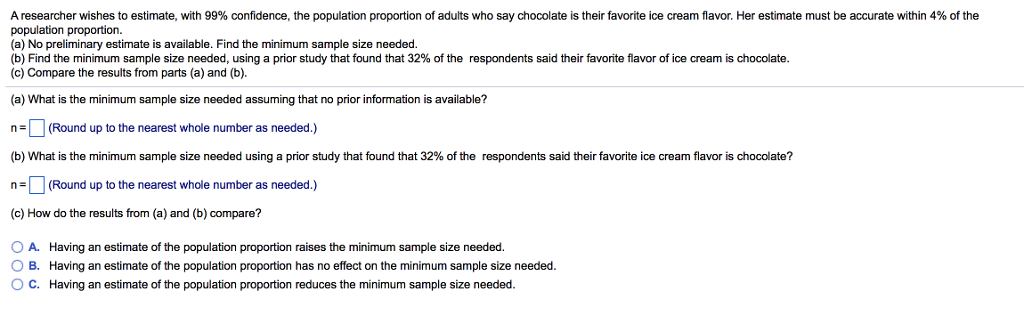This image displays a webpage featuring a statistics problem related to estimating the population proportion of adults who say chocolate is their favorite ice cream flavor. The background of the webpage is entirely white, creating a clean and distraction-free environment for the focal content. 

At the top of the page, the text reads: "A researcher wishes to estimate with 99% confidence the population proportion of adults who say chocolate is their favorite ice cream flavor. Her estimate must be accurate within 4% of the population proportion." 

Below this introductory statement are three distinct questions labeled A, B, and C:
- **A:** "No preliminary estimate is available. Find the minimum sample size needed."
- **B:** "Find the minimum sample size needed using a prior study that found 32% of the respondents said their favorite flavor of ice cream is chocolate."
- **C:** "Compare the results from parts A and B."

Further down the page, there are three selectable bubbles corresponding to different statements about the effect of having an estimate of the population proportion on the minimum sample size needed:
1. "Having an estimate of the population proportion raises the minimum sample size needed."
2. "Having an estimate of the population proportion has no effect on the minimum sample size needed."
3. "Having an estimate of the population proportion reduces the minimum sample size needed."

This layout provides users with a clear, step-by-step approach to tackling the statistical problem presented, complete with options to choose from for interactive learning.